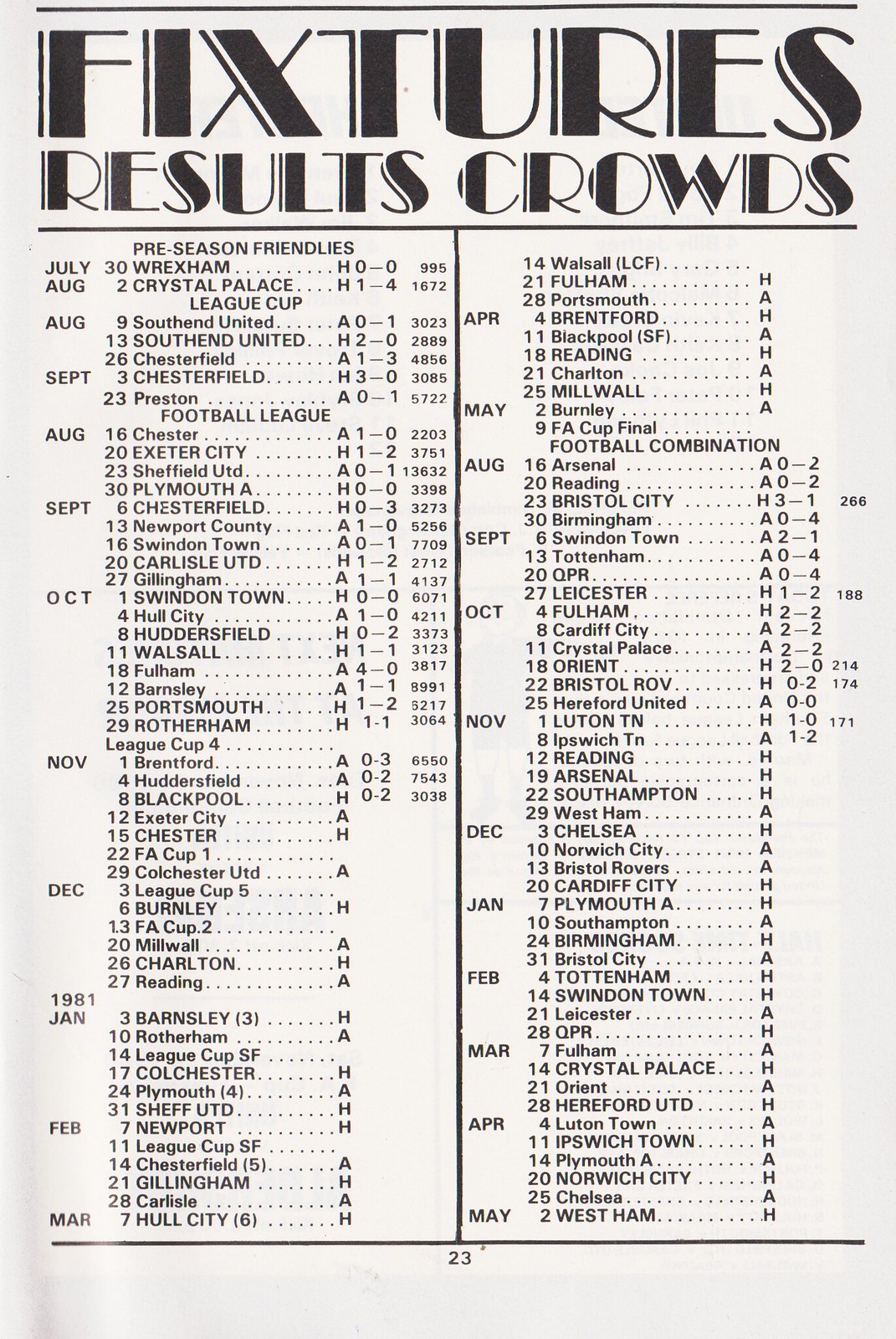The image appears to be a page from a sports program or magazine, specifically showcasing "FIXTURES, RESULTS, CROWDS" in bold, capital letters at the top. The content is organized into two main sections with dates and game results spanning from July in the left column to May of the following year in the right column. Each entry lists a date, a team, and the game's result, such as "July 30th: Wrexham, H 0-0" and "August 2nd: Crystal Palace, H 1-4." The entries are compact and numerous, indicating a comprehensive record of match outcomes over several months. There is an indication of the document being from a specific season, with pre-season friendlies possibly mentioned. The layout is crowded with data, making it somewhat challenging to discern at a glance, but it effectively captures the detailed results of numerous matches in black and white.